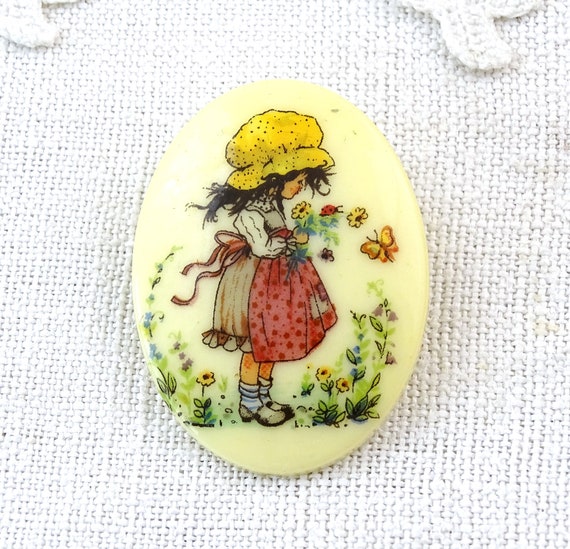The image features a detailed depiction of a little girl painted on an oval-shaped object, possibly a badge, pin, or decorative piece, which is resting on a light-colored knit cloth, suggesting it might be a tablecloth or similar fabric. The girl, who appears to be in an old-fashioned, "Holly Hobbie"-style attire, is dressed in a yellow bonnet and a tan dress with a red apron. She has dark, long hair and is wearing slouchy blue socks paired with clog-like black shoes. She stands in a garden filled with various flowers and plants, looking over her shoulder while holding a flower. Nearby, there are insects, including a ladybug close to her face and a butterfly to the right of her. The strings of her apron flow gently behind her, adding a dynamic element to the serene and nostalgic scene.